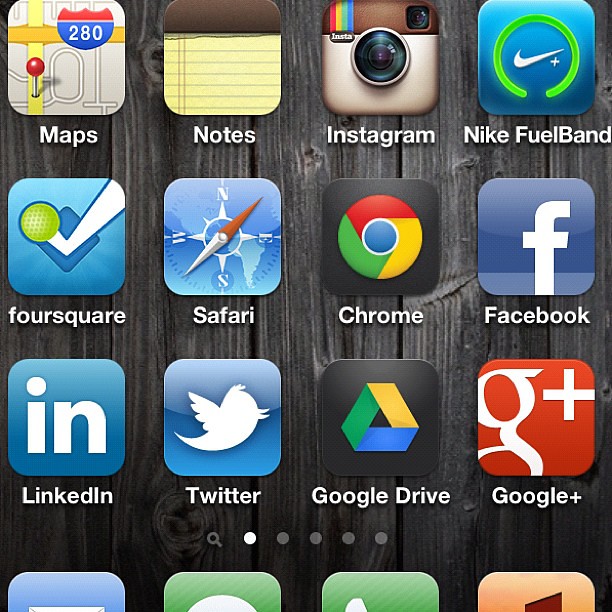The image depicts a screen displaying a variety of app icons arranged in a grid format. The exact device is uncertain, as it could be the screen of a phone, tablet, or computer. Starting from the top row, the visible app icons include Maps, Notes, Instagram, Nike, and FuelBand. The second row features Foursquare, Safari, Chrome, and Facebook. The third row presents LinkedIn, Twitter, Google Drive, and Google Plus. There are additional icons visible at the bottom of the screen, but they are partially obscured and not fully readable. The background of the screen has a subtle, textured grayish wood design, adding a distinct yet understated aesthetic to the arrangement of the app icons.